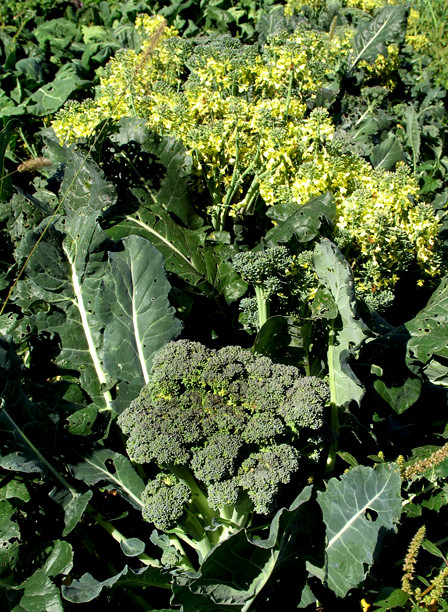The photograph, presented in a vertically rectangular frame, showcases a close-up view of a garden filled with broccoli plants under bright, sunny lighting, casting both illuminated and shadowed areas. The garden appears to be past its prime, with several indicators of neglect. Prominent dark green leaves are seen throughout, many showing signs of insect damage with visible holes. In the lower central portion of the image, there is a large broccoli head, its color blending with the surrounding leaves but exhibiting a textured, almost bushy appearance. Unfortunately, this particular broccoli head appears brown and nearly rotting. The upper portion of the photograph is dominated by a cluster of bright yellow and white flowers, signifying that the broccoli has gone to seed. The presence of scattered grasses and weeds further emphasizes the untended state of the garden.